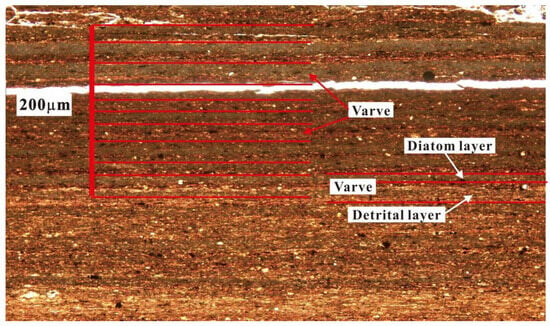This image depicts a close-up view of stratified soil or sediment layers, primarily in varying shades of brown. The layers exhibit different hues, with darker brown at the top transitioning to lighter brown towards the bottom. A prominent white horizontal line crosses near the top quarter of the image, marked with "200 UM" in black text. Multiple thin red lines horizontally dissect the brown surface, each accompanied by labels and arrows indicating different layers. Notably, the labels include "varve," "diatom layer," and "detrital layer," each designated by red lines and arrows. Additionally, a bold vertical red line at the top of the image is emphasized by two red arrows, also marked as "varve."